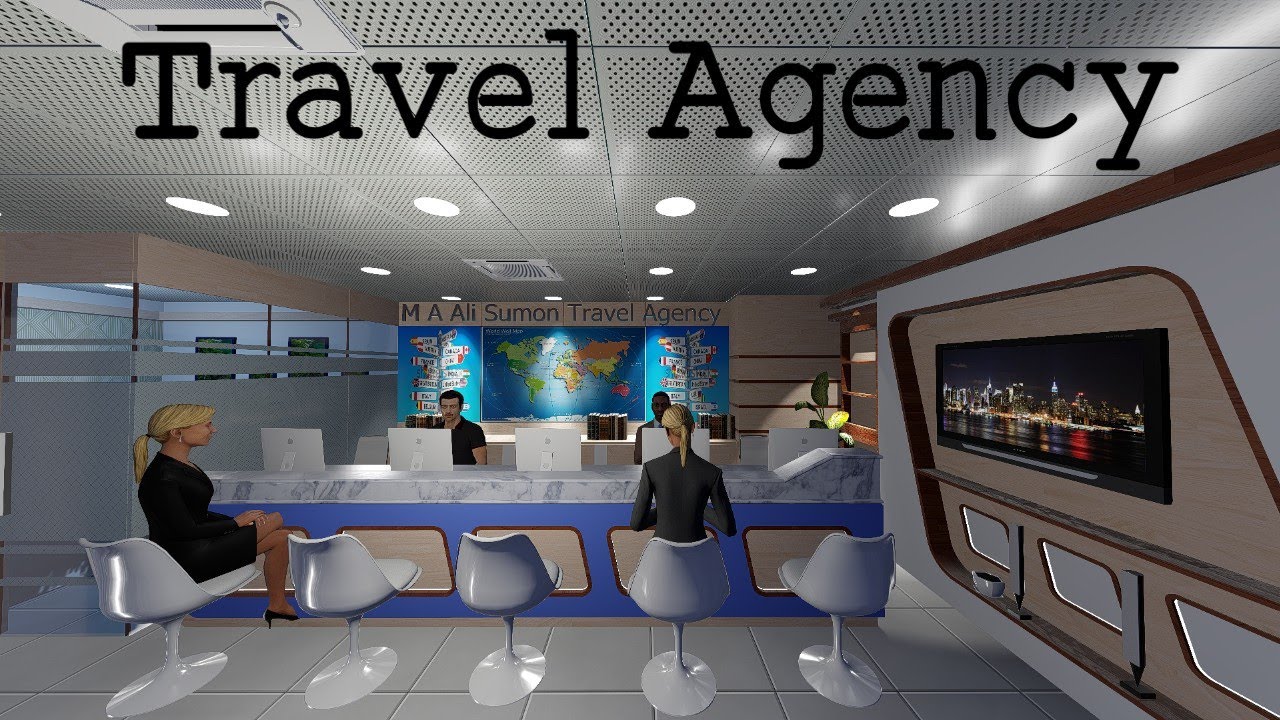The image depicts a digital 3D rendering of a modern travel agency’s reception area or common workspace. The flooring consists of large, gray square tiles, adding a sleek, professional ambiance. Prominently displayed at the top of the scene, in bold black letters, is the label "Travel Agency". Below this, in the far background, a white wall features a massive, floor-to-ceiling three-panel map showcasing the continents of the world, with "M.A. Ali Suman Travel Agency" written across it in blue text. 

In the foreground, there are five futuristic white plastic swivel chairs with single leg supports and round bases. Two of the chairs are occupied by women, one seated in the first chair and the other in the fourth. They appear engaged in conversation with two men seated on the opposite side of a sleek, white marble counter, working at white laptop computers. Computer monitors are set up in front of each chair. 

To the right, built into the otherwise white wall, is a flat-screen television displaying a video or image of a large city skyline at night, adding a dynamic visual element to the space. The ceiling consists of a white drop-down design outfitted with lights, completing the modern and sophisticated aesthetic of the travel agency environment.